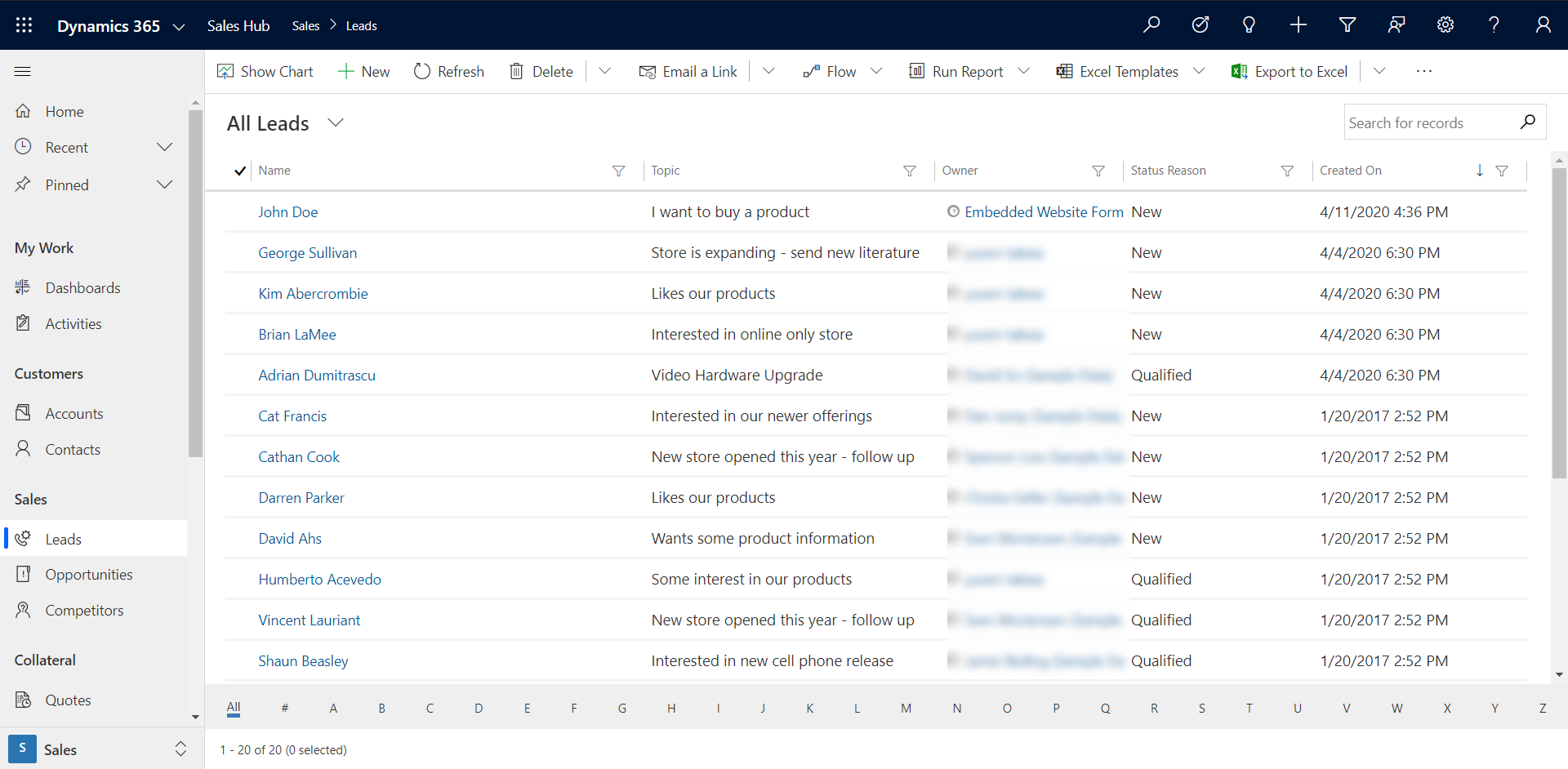**Screenshot of the Sales Hub Interface in Dynamics 365**

The screenshot features the Dynamics 365 Sales Hub interface, showcasing a clean, white page with black text. It's primarily focused on the "Leads" section. The top navigation bar includes various icons: a compass, light bulb, plus sign, magnifying glass (flashlight), silhouette of a body (twice), settings gear, question mark, and more. Main options available are "Show chart," "New," "Refresh," "Delete," "Email a Link," "Flow," "Run Report," "Excel Templates," "Export to Excel," and "Search for Records."

The page displayed is "All Leads," listing names such as John Doe, George Sullivan, Kim Abercrombie, Brian Lemieux, Adrian Dimitra, Sue Cat, Francis Cook, Catherine Parker, David Darren, Humberto Beasley, Acevedo Sean, and Vincent Doe Laurent. Detailed lead information such as statuses and actions include: "Expanding to buy a product like our products and new literature," "Upgrade interested," "Online store only," "New store open this year," "Follow up video hardware," "Wants some product information," "Interested in cell phone release," and multiple leads marked as "Qualified" and "New."

The interface effectively consolidates essential elements required for managing sales leads, emphasizing actionable insights and providing numerous tools to streamline sales processes. The captured time indicates 4:30 PM, offering a snapshot of the active tasks and ongoing lead management efforts.